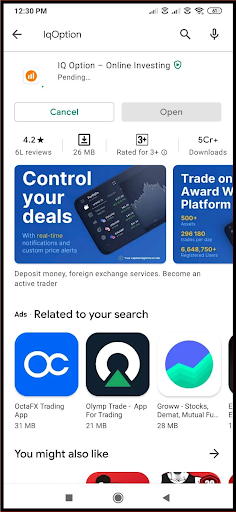This image is a screenshot taken from a cell phone at 12:30 PM, as indicated by the timestamp in the top left corner. The screen displays various icons at the top, showing a battery level at 60%. Below this notification area, on the left side of the screen, there's a back arrow icon labeled "IQ Option," while on the right side of the screen, there is a magnifying glass icon for search and a microphone icon for voice commands.

Further down, the main portion of the screen features a prominent orange circle with white bars at its center, encased in a white square. This is accompanied by the text "IQ Option Online Investing Plus," followed by the word "Pending." Next to this information, there are two buttons: one for "Cancel" and another for "Open."

Moving down the page, it indicates a rating of 4.2 stars based on 61 reviews. The app's download size is specified as 126 megabytes, and it is rated for users aged 3 and above. Additional content on the screen includes advertisements with messages like "Control your deals, trade on award," and a section titled "Related to your search" towards the bottom of the screen.